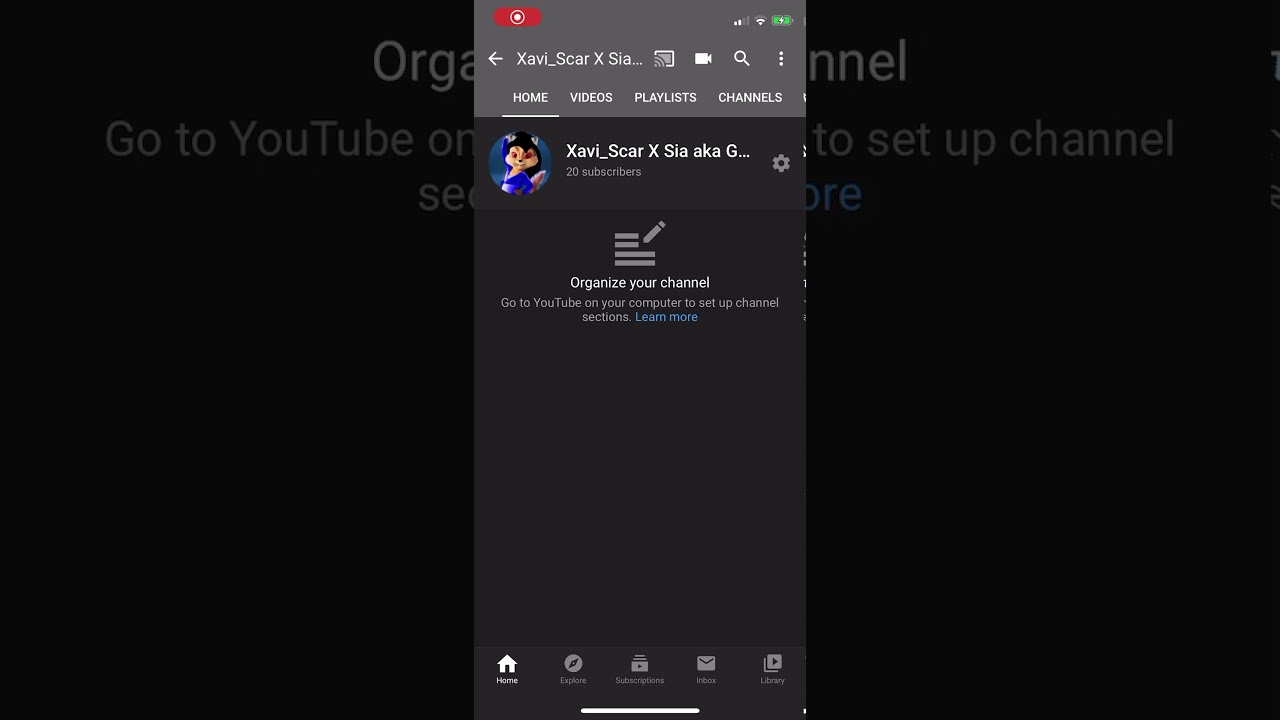This image features a landscape-oriented screenshot with a smaller portrait-oriented mobile phone screenshot centered within it. The background is a black screen displaying partially visible grey text divided by the foreground screenshot. On the left side, the text reads "Orga," followed by "Go to YouTube On," while on the right side, it states "To set up channel."

The mobile phone screenshot in the foreground is the focal point of the image. It displays an app interface in greyscale tones. The top bar is light grey with white text, indicating the user's profile name: "Xavi_ScarXSia." Adjacent to the left-facing arrow icon, which signifies the back button, there are different utility icons on the right: screen sharing, video, search, and a menu represented by three vertical dots.

Beneath this top bar, there are four selectable tabs: Home, Videos, Playlists, and Channels. The Home tab is currently selected, as indicated by the white underline. Directly under these tabs lies a dark grey section featuring a circular profile picture of a cartoon chipmunk with red eyes, clad in a black outfit and hood, situated at the top left. To the right of this profile image, the white text reads "Xavi_ScarXSia aka G…," and below, in smaller light grey text, it states "20 subscribers," with a settings icon aligned further to the right.

Occupying the majority of the screenshot beneath the profile information, a darker grey background presents further instructions. It shows the message "Organize your channel" in light grey text at the top. Following this is smaller text instructing, "Go to YouTube on your computer to set up channel sections," and a clickable "Learn more" link in blue text. Central to this lower section, there is an icon with two short lines and a pen symbol next to it, followed by two longer lines beneath.

The bottom of the screenshot features a menu bar with white icons and text, arranged from left to right as follows: Home (house icon), Explore (compass icon), Subscriptions (draw icon), Inbox (envelope icon), and Library (play icon).

Overall, this detailed caption comprehensively describes the layout and elements present in the dual-screenshot image.